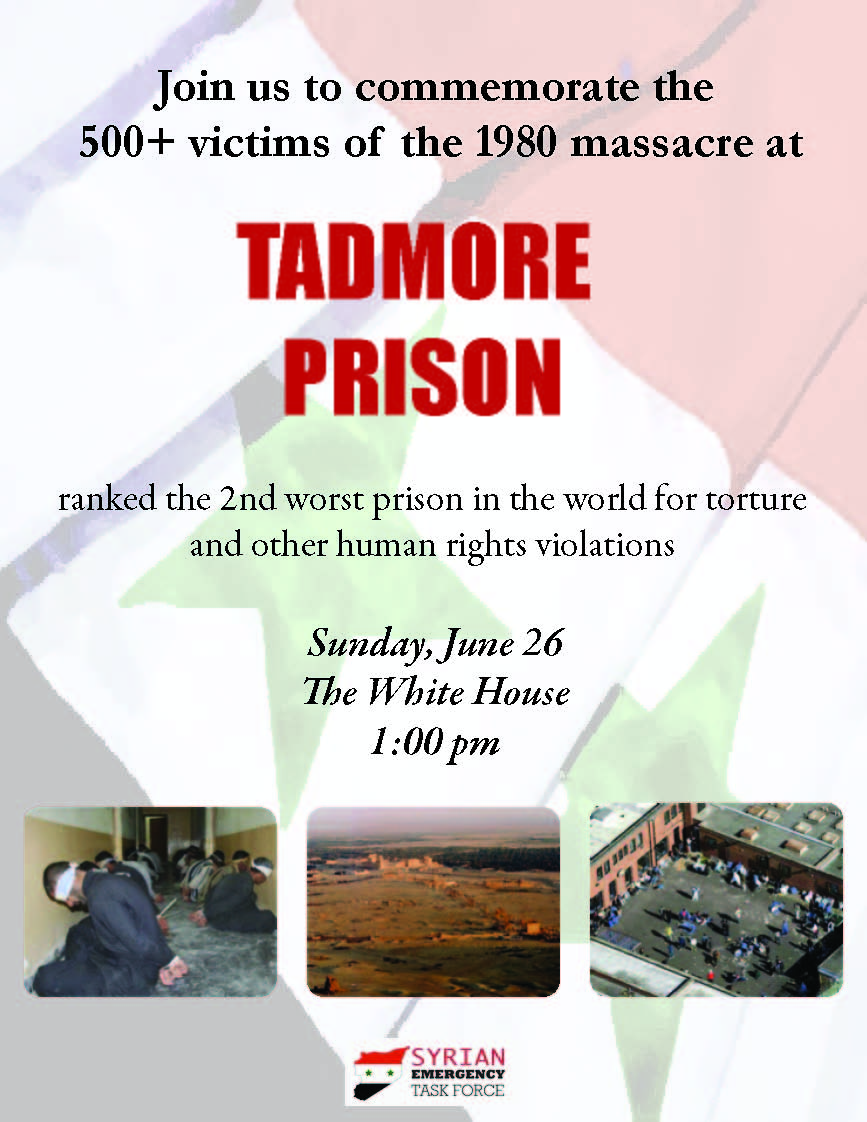The advertisement banner for the event features a background of a waving flag, distinctively colored red at the top, white in the middle, gray in the bottom left, with green stars. Dominantly displayed in black text at the top, it says, "Join us to commemorate the 500 plus victims of the 1980 massacre at," followed by "Tadmore Prison" in bold, large red text. Below this, black text states, "Ranked the second worst prison in the world for torture and other human rights violations." An italicized line in black text announces, "Sunday, June 26th, the White House, 1 p.m."

At the bottom of the banner are three poignant pictures. The leftmost image depicts prisoners kneeling on the ground with their heads bowed and blindfolded, their hands tied behind their backs, dressed in blue uniforms. The central image offers an aerial shot of the prison from a significant distance, while the rightmost image provides a closer, above-ground view of the prison yard.

Beneath these images, a symbol outlines the country of Syria, with the same color scheme as the flag: red on top, white in the middle with green stars, and black at the bottom. The text near the symbol reads, "Syrian Emergency Task Force."